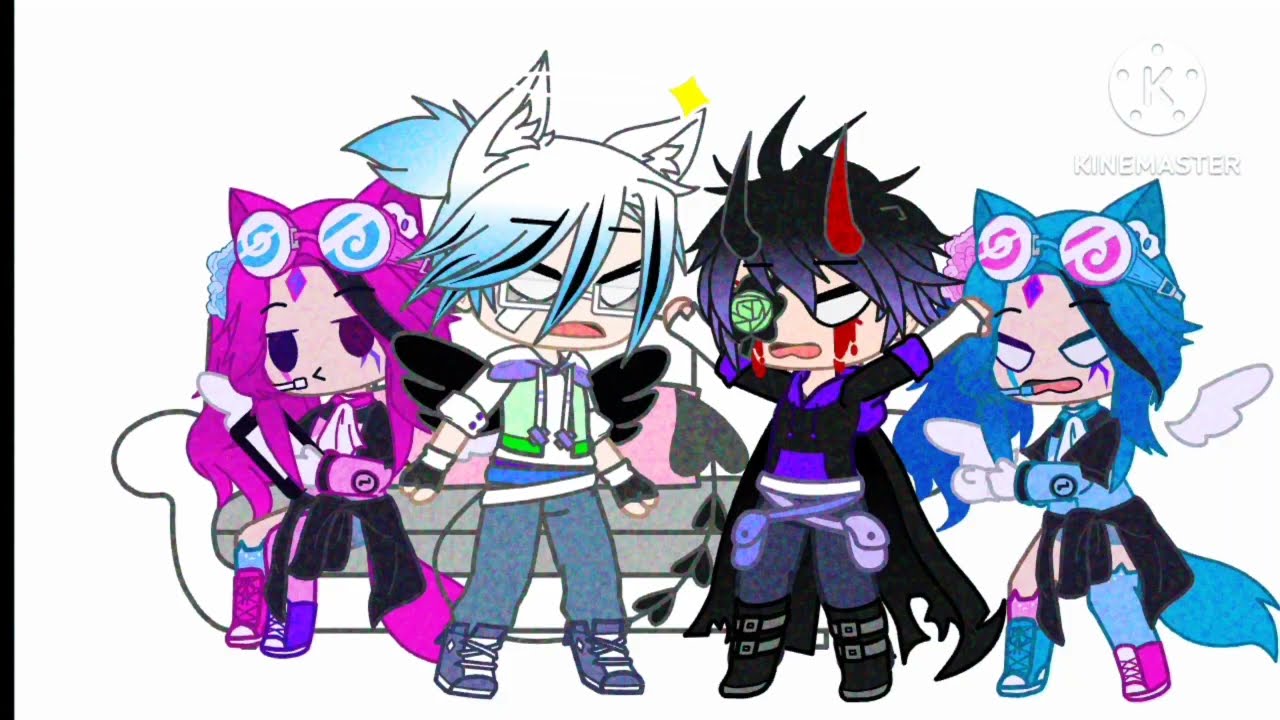This image features four human-like anime-style characters against a white background. There's a distinct logo in the top right corner, a letter "K" within a circle, labeled "KINEMASTER" below it. All characters have white eyes and are dressed in modern trench coats with sneakers of various colors. 

Starting from the left, the character has dark pink hair styled with a pink fox hood, white goggles perched on her forehead, a microphone, and a black robe. She is seated on a gray sofa with white cushions. 

Next to her is a character with turquoise hair and light blue fox ears, donning a turquoise tail, black wings, a blue shirt or blazer, and a black sweat-hooded sweatshirt tied around her waist.

Moving to the right, the third character sports white and blue hair with white fox ears, white-framed glasses, a green, purple, and white top, blue jeans, and purple shoes. 

The fourth character on the far right has dark purple hair with red and black horns, a green eye patch over her right eye, blood marks under her eyes, black eyeliner, and a predominantly purple and black outfit. She is primarily color-coded in pink, blue, and purple hues. 

This intricate blend of colors and styles gives each character a unique and vivid appearance, enriched by detailed accessories and hairstyles.